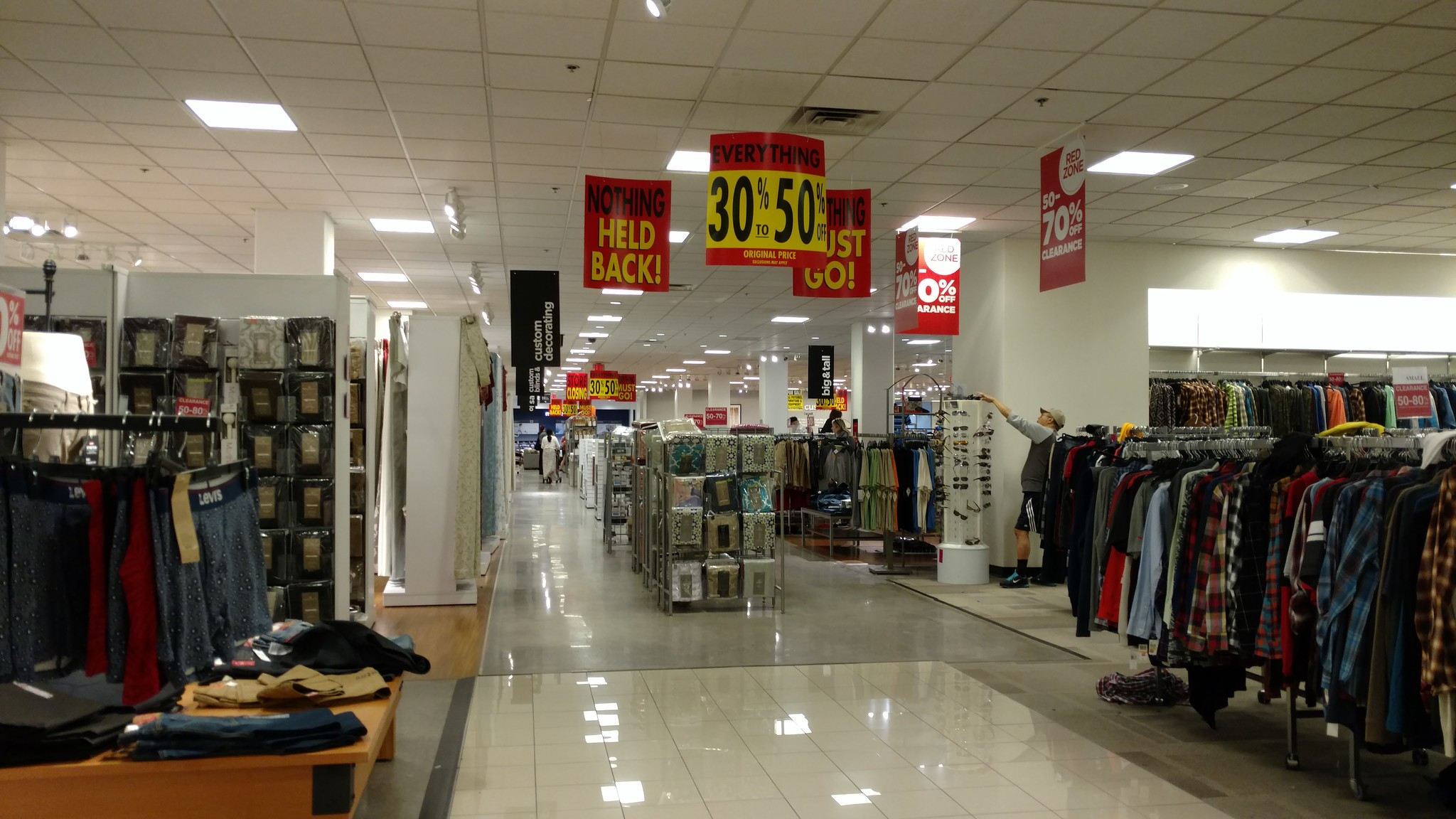The image depicts the interior of a department store, reminiscent of a Macy's, where a significant clearance sale is in progress. The scene is looking directly down a wide aisle lined with various apparel and household items. The store's floor is tiled with a clean white, gray, and beige pattern, reflecting the abundant fluorescent lighting from the ceiling's white drop tiles with gray framing. 

To the left, there are shelves displaying folded jeans and pants on a brown wooden display case, alongside boxer shorts hanging on racks. Prominently, a section of Levi's jeans is visible. To the right, an array of men's clothing, including dense rows of plaid long-sleeve shirts, fill the racks. A man dressed in shorts, a long-sleeved shirt or sweater, and a hat is seen reaching for an item on top of a display case, which appears to have sunglasses on it.

Suspended from the ceiling, striking red, yellow, and white signs declare various discounts such as "Nothing Held Back", "Everything 30-50% Off Original Price", "Everything Must Go", and "Red Zone 50-70% Off Clearance". The shelves in the center aisle have assorted items, including what appears to be sheets. Various shoppers are seen moving through the aisles, adding to the bustling atmosphere of the store, eager to take advantage of the substantial discounts.